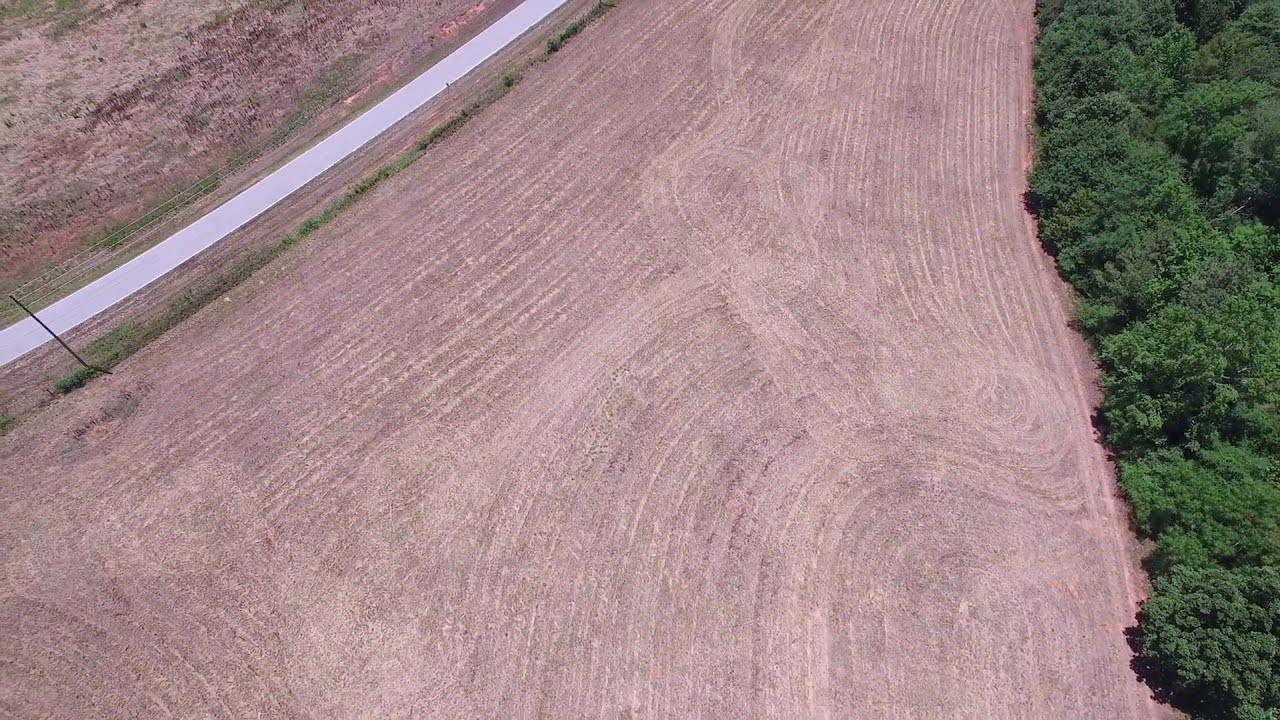The image depicts an outdoor scene from a top-down, bird's-eye perspective, showcasing a varied landscape. The right hand side features a dense cluster of trees with vibrant green leaves, occupying about an eighth of the frame. In contrast, the left side presents a starkly different view with a predominantly dry, dull brown patch of grass, interspersed with irregular green areas. Adjacent to this grass, there's a small, white path that appears unoccupied. Dominating the center and most of the image is a vast, brown field exhibiting numerous lines from plowing or sowing, some of which are straight, while others curve or circle. A plain, light gray cement road winds from the middle left to near the top center of the image, cutting through the scene. To the left of this road lies another dirt area, unmaintained and sprinkled with gray, brown, green, and red weeds, indicating neglect. Additionally, there is one visible electrical line pole towards the left middle of the image.